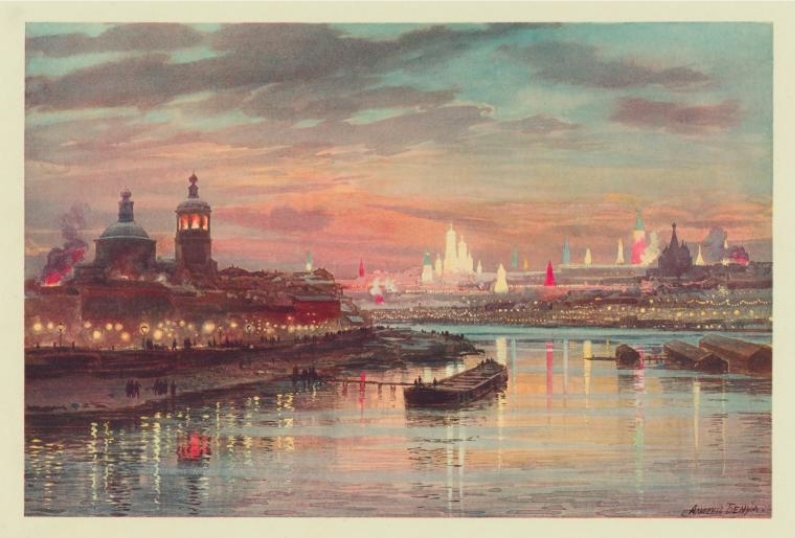This detailed oil painting, titled "Coronation of Nicholas II, Illuminations in Moscow" by Albert Benoit, created in 1896, captures a captivating evening river scene in Russia, illuminated under a pink and blue sunset sky with dramatic clouds. The painting, set in a landscape orientation with an off-white border, prominently features a body of water populated by a few boats and a central barge. On the right side, the water laps against a coastal area dotted with buildings in gray, white, and red simplistic shapes. To the left, the shoreline glows with a row of lights, enhancing the silhouettes of numerous structures, including high towers and domes adorned with ornamental crosses. Some buildings appear almost illuminated with lights, contributing to the vibrant nightlife atmosphere. Billowing smoke and darker shadows are present on the periphery, adding depth to the twilight setting. The artist's signature is discernible at the bottom right, and the painting is rendered in a palette of blue, gray, tan, red, orange, pink, yellow, light blue, brown, and black, embodying the Russian Impressionism style.